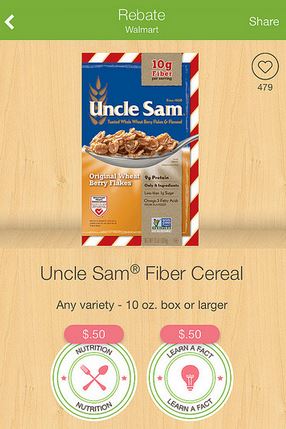This image captures a digital device, likely a phone or tablet, displaying a webpage featuring details about a rebate offer from Walmart. The webpage header includes the word "Rebate" in white letters on a green bar, with the option to "Share" located to the right.

Prominently displayed in the center is a box of Uncle Sam cereal. The top half of the cereal box is blue while the bottom half is yellow, with a red and white striped border that evokes the design of the American flag. The box reads "Uncle Sam" in bold white letters. The packaging is placed on a light-colored wooden surface, which serves as the background for the image.

At the bottom of the image, the background continues with the same light wood texture, and text in dark brown reads "Uncle Sam Fiber Cereal" followed by "Any variety 10 ounce box or larger."

Two informational circles are displayed below this text. The circle on the left mentions "50 cents Nutrition Nutrition" along with an icon of a fork and spoon in pink. The circle on the right also mentions "50 cents" and "Learn a Fact," accompanied by a pink light bulb icon in the center.